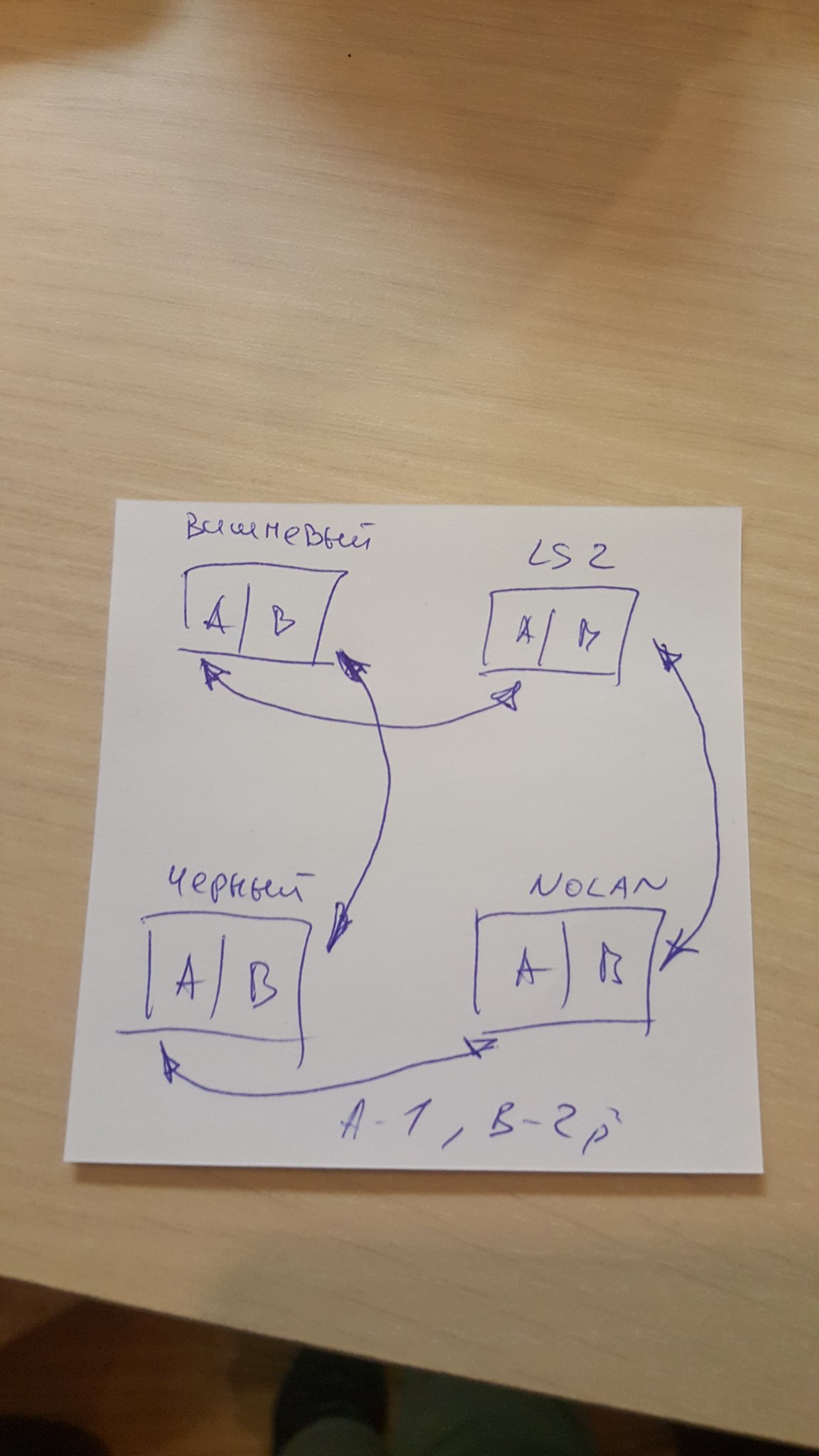In this image, a square piece of paper lies on a light tan wooden table, positioned slightly tilted to the left near the bottom of the frame. The paper features a variety of labeled sections and arrows indicating connections between them. In the upper left-hand corner, there is a rectangle divided into two squares marked "A" and "B," with a word written above them in cursive, possibly a name, though it is not legible. To the right of this section, there is another box labeled "LS2," also divided into two sections marked "A" and "B," connected by arrows pointing back and forth. 

Further down, there are two more rectangles with divided squares. The bottom left rectangle, labeled with an unreadable cursive word, is also marked "A" and "B" and has an arrow connecting it bidirectionally to the section above it. To the right, another rectangle is identified with the label "Nolan" and is similarly divided into "A" and "B." This rectangle has an arrow linking it bidirectionally to the section above labeled "LS2," and both bottom rectangles also have arrows pointing back and forth to each other. The bottom of the paper features the notations "A-1" and "B2P."